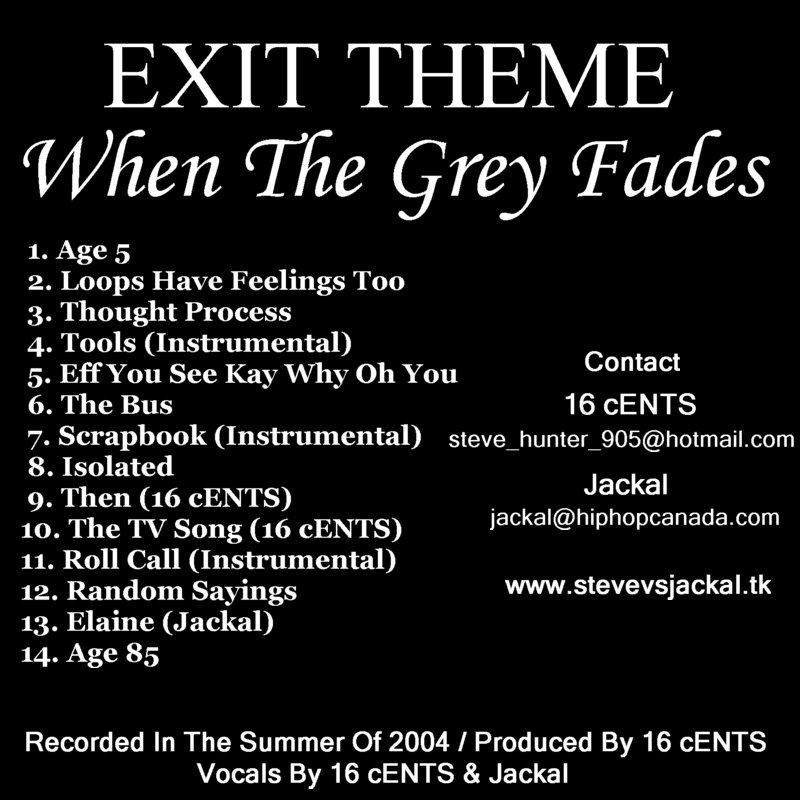This image appears to be the album cover for "Exit Theme: When the Gray Fades" by artists Sixteen Cents and Jackal. The cover features white text on a black background, with the title "Exit Theme" in a prominent, Times New Roman-style font, while "When the Gray Fades" is written in a more abstract and flowy font. Below the title, aligned on the left side, is a list of 14 song titles, including:

1. Age 5,
2. Loops Have Feelings 2,
3. Thought Process,
4. Tools (Instrumental),
5. F-U-C-K-Y-O-U,
6. The Bus,
7. Scrapbook (Instrumental),
8. Isolated,
9. Done by Sixteen Cents,
10. The TV Song by Sixteen Cents,
11. Roll Call (Instrumental),
12. Random Sayings,
13. Elaine Jackal,
14. Age 85.

On the right side, the cover features additional white text that provides contact information: "Contact: Sixteen Cents, Steve Hunter 905 at hotmail.com, Jackal at hiphopcanada.com." Below this, it states, "Recorded in the summer of 2004, produced by Sixteen Cents. Vocals by Sixteen Cents and Jackal." This detailed listing and information capture the essence of the album's presentation, making it clear and informative.